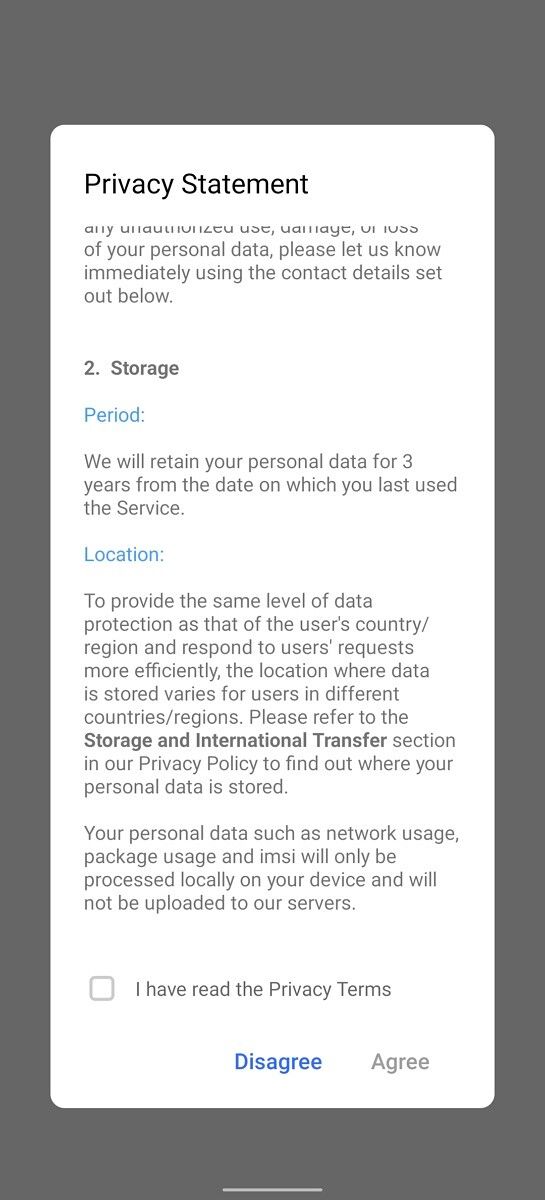Screenshot of a Privacy Statement Pop-Up on a Mobile Device

The screenshot displays a privacy statement pop-up on a mobile device. The background is a medium dark gray, accentuating the lighter colored pop-up window, which is a white or very light gray with rounded edges. The text within the pop-up is dark gray, maintaining readability against the light background. Links and categories within the statement are highlighted in various shades of blue and a greenish-blue, with the "Disagree" link notably appearing in a distinct shade of blue to indicate its interactive nature.

At the bottom of the pop-up, there are prominent "Agree" and "Disagree" buttons, allowing users to make a choice. A check box labeled "I have read the privacy terms" is present just above these buttons, though it remains unchecked. The user seems to be scrolling through the privacy policy text, which is partially visible.

The first paragraph introduces the privacy terms, while the subsequent paragraphs detail specific aspects like data storage and location. Notably, it mentions that personal data will be retained for three years from the last use of the service and emphasizes compliance with the user's local data protection regulations. The location of data storage varies depending on the user's region, and there is a reference to the "Storage and International Transfer" section for more details. Additionally, it assures that personal data such as network usage, package usage, and IMSI will only be processed locally on the user's device and will not be uploaded to the server.

The comprehensive layout and design aim to ensure full disclosure and offer the user various options to interact with the privacy terms, ultimately leading to an informed decision.